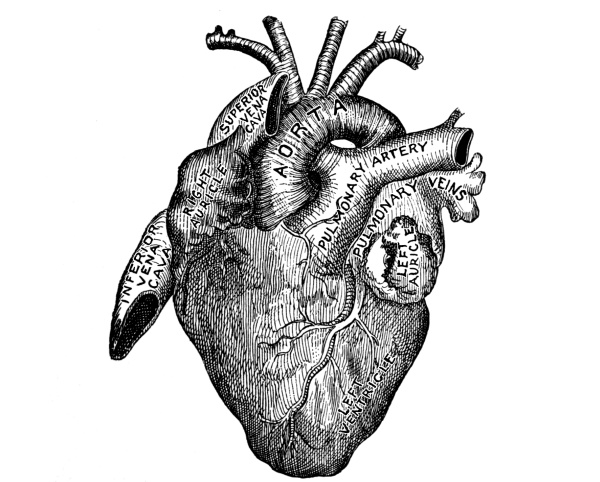This image is a detailed black and white medical illustration of an anatomical heart, seemingly drawn with a fine point pen on a white or transparent background. The heart is centrally positioned within a square frame, and it features clearly labeled parts including the inferior and superior vena cava, right auricle, aorta, pulmonary artery, pulmonary veins, left auricle, and left ventricle. The drawing meticulously includes details such as open and curved tubes, with some areas highlighted in black where the openings are depicted. It showcases the intricate network of veins and arteries, resembling real anatomical features rather than symbolic representations, and highlights the impressive complexity of the organ.